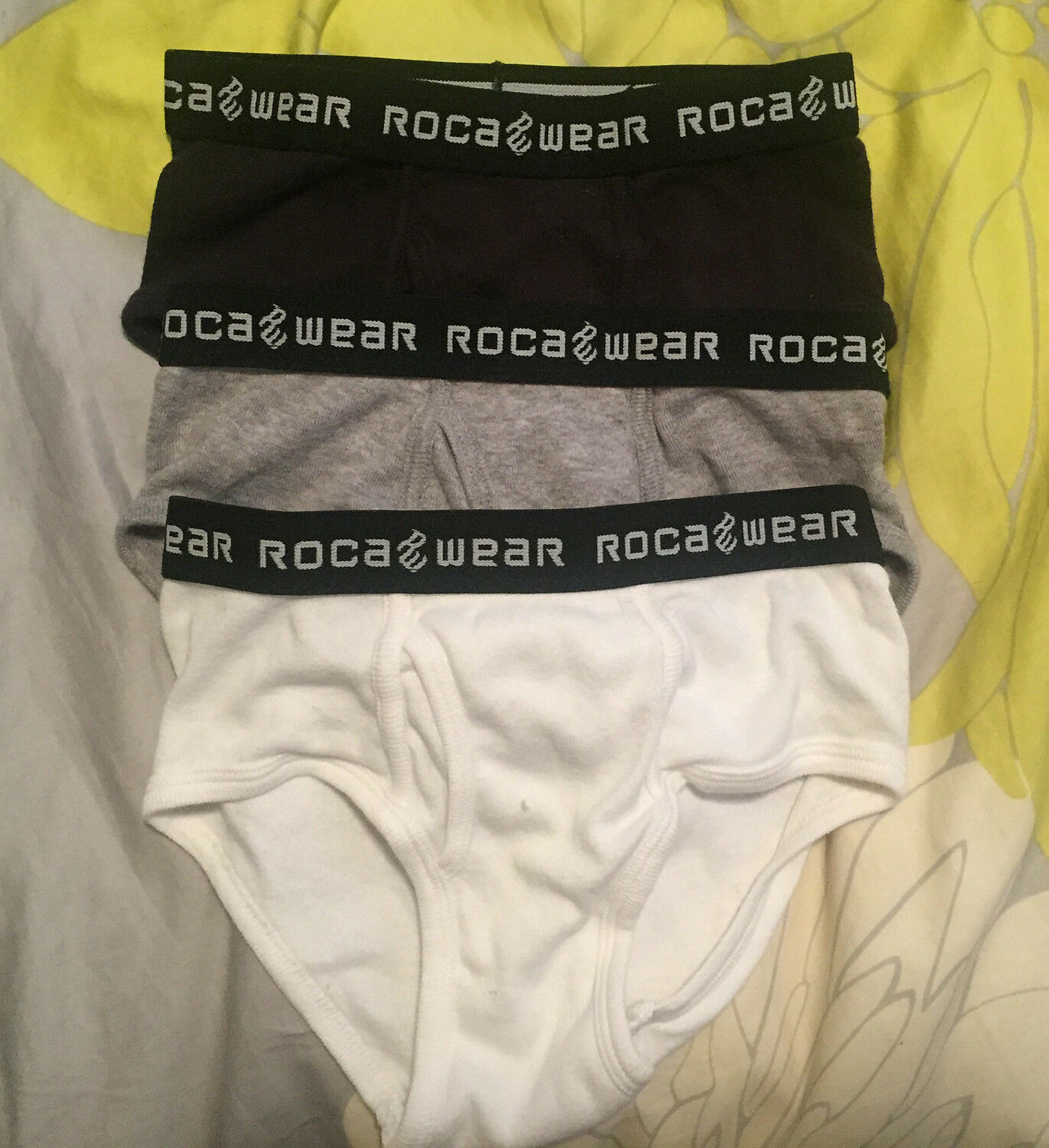The image depicts three pairs of men's cotton briefs, each displaying a black elastic waistband emblazoned with the brand "ROCAWEAR" and the "RW" logo. The briefs are arranged in a layered fashion with the black pair on top, followed by a heather gray pair in the middle, and a white pair at the bottom. The waistband lettering is a grayish color. These soft and short-styled briefs are laid out on what appears to be a bed sheet adorned with a floral design featuring cream petals and yellow flowers, with gray floral prints clustering in the lower left corner. The bed sheet's background transitions from predominantly white in the bottom right to mostly gray on the left side and yellow towards the top right, creating a vibrant, textured backdrop for the underwear display.